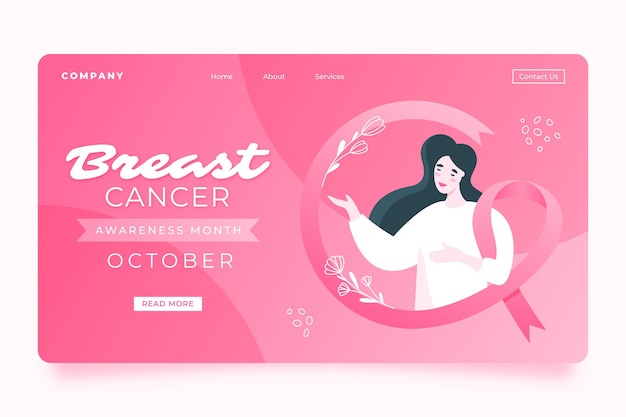The image displays a clean, white background with a prominent pink rectangle in the center, featuring rounded corners. Within the rectangle are navigation headings that read: "Company," "Home," "About," "Services," and "Contact Us." Positioned to the left of the rectangle, the text highlights "Breast Cancer Awareness Month," "October," and "Read More." Notably, the word "Breast" is elegantly scripted in white cursive font, while "Cancer" and "Awareness Month" are in bold, all-capital, white letters. The phrase "Awareness Month" is framed inside a pink ribbon, symbolizing the cause. The word "October" is also in bold, uppercase letters.

To the right, an illustration depicts a flowing pink ribbon. It starts with a 'C' shape at the top, loops at the bottom, forming the classic breast cancer awareness ribbon. Embedded within the ribbon's lower loop is an illustration of a woman with long black hair, wearing a long sleeve white top. Her left arm is gracefully threaded through the loop of the ribbon, and her right hand is reaching upward, her face adorned with a gentle smile. Surrounding the ribbon are delicate line drawings of flowers, adding an elegant touch. The entire composition is devoid of animals, keeping the focus on the awareness and support for breast cancer.